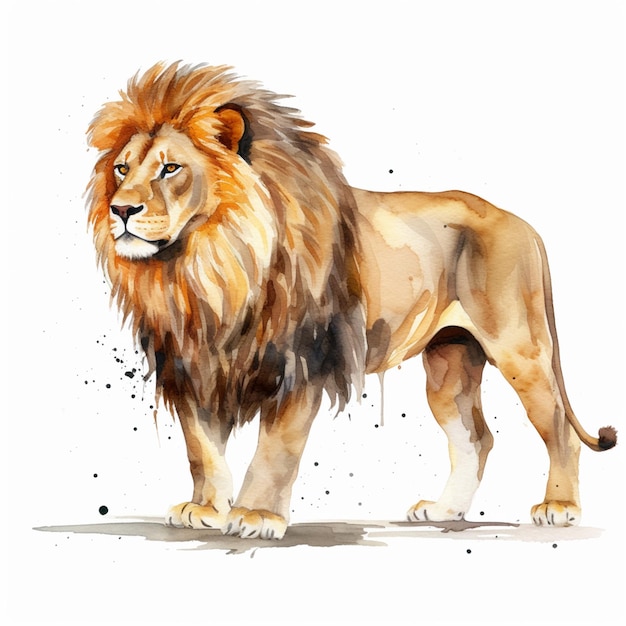This detailed watercolor painting depicts a powerful male lion standing on all fours, facing slightly left towards the camera. The lion's piercing yellow eyes and closed mouth, paired with its majestic, full mane, evoke a sense of fierceness. The mane transitions from medium brown at the top to dark brown and black at the bottom, featuring some white around the face and brown behind the ears. The lion's light brown body, accented with shades of black, stands on a shaded gray and light gray surface. Its thick legs are a light brown, ending in white paws, and its long, narrow tail, also light brown, curves up slightly with a dark brown fuzzy tip. The image is set against a stark white background, with black paint splatters scattered beneath the lion and a few above its back, enhancing the artistic, slightly cartoonish yet realistic feel of the watercolor painting.